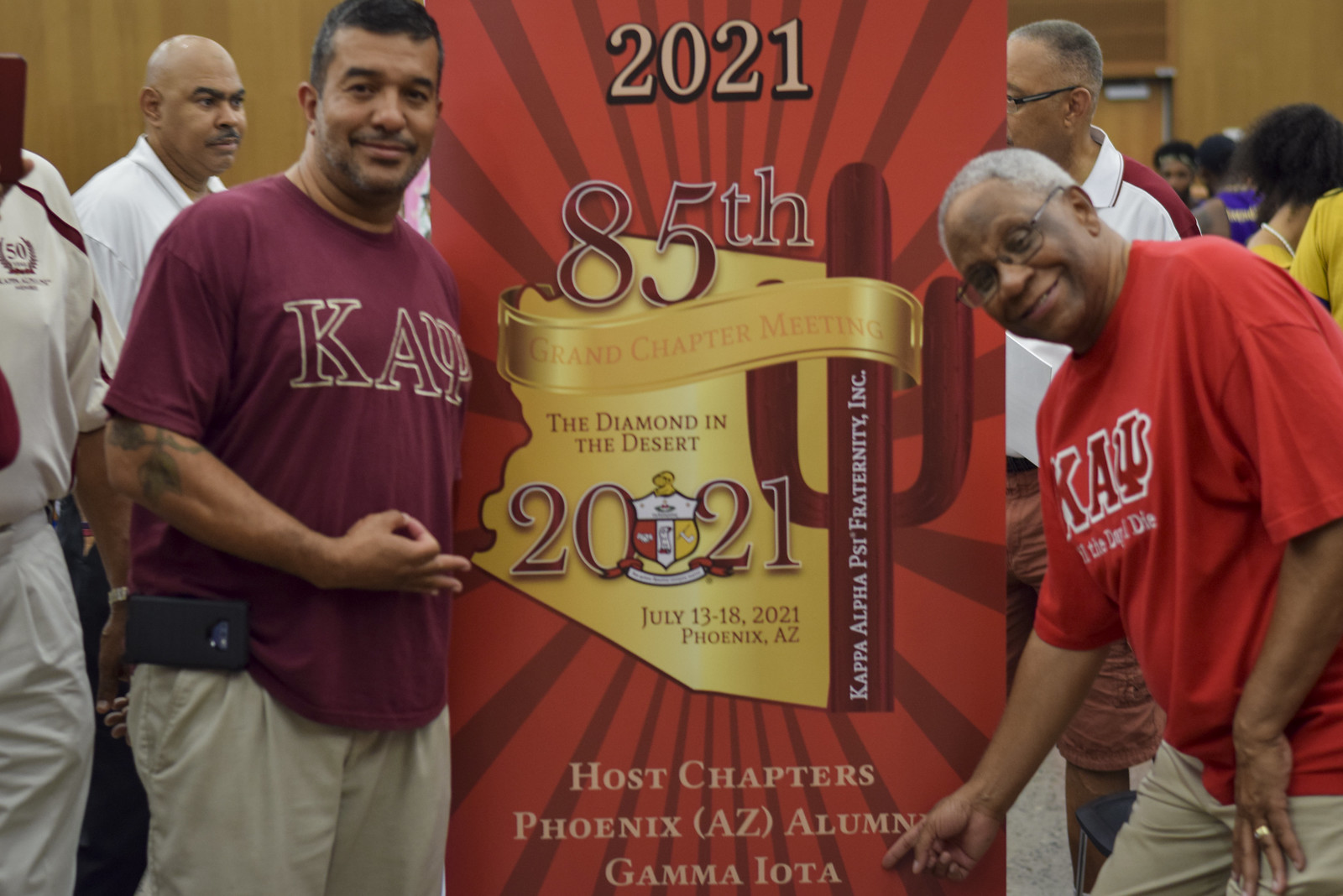In the image, two men are prominently featured in front of a red banner. The larger man on the left, an older black gentleman, wears a maroon shirt with the letters "K-A" and a pitchfork-like symbol, along with beige pants. His right arm is near his stomach, forming a circle with his hand. The man on the right sports a matching shirt in red, also emblazoned with the same "K-A" letters and pitchfork design. He too is holding his right hand in a circular gesture. The banner behind them is predominantly red and reads "2021 85th Grand Chapter Meeting: The Diamond in the Desert, July 13-18, 2021, Phoenix, Arizona." It features a gold emblem and the host chapters listed as Phoenix, AZ Alumni and Gamma Iota. Additionally, the backdrop includes an outline of the state of Arizona and a red cactus. Both men appear to be posing proudly, highlighting their affiliation with the Kappa Alpha Psi Fraternity Incorporated.